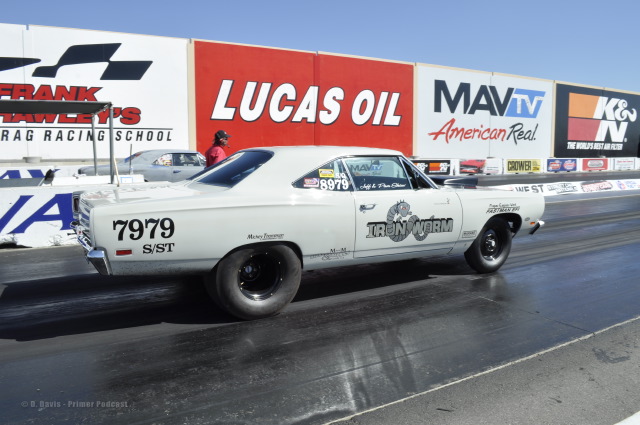This image features a white, old-school race car on a slightly wet raceway, showcasing athletic design elements typical of sports cars. The car prominently displays the number 7979 on its rear. On the side door, there's a distinctive logo of an intertwined worm labeled "Iron Worm." The car is equipped with special racing tires, enhancing its competitive appearance. Numerous sponsors’ logos adorn the vehicle and the surrounding area, including Lucas Oil, MAV TV American Real, K&N, and Frank’s Drag Racing School. Additionally, a large white and red sign in the background displays various advertisements. A man in an orange shirt and baseball cap stands behind the car, and there is a watermark towards the bottom left of the image reading "D. Davis Premiere Podcast." The background also features a blue sky in the upper right corner.